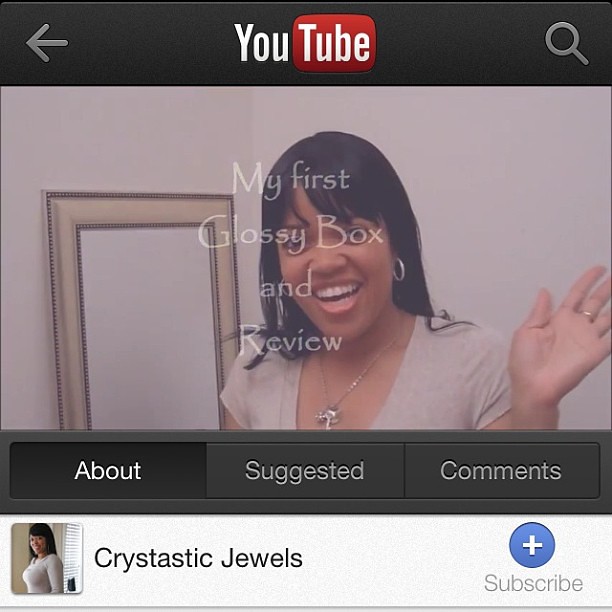This image captures an old YouTube page from the Christastic Jewels channel, showcasing the classic YouTube layout. At the top, the recognizable YouTube logo sits inside a red square. In the main frame, an African-American woman with straight black hair and bangs is seen smiling and waving to the camera. She is wearing small silver hoop earrings, a necklace, a white v-neck t-shirt, and a ring on her middle finger. In the background, a large mirror prominently features. Overlaying her face is white text stating "My First Glossy Box in Review," indicating the video title. Below the main video screen, there are several clickable buttons labeled "About," "Suggested," and "Comments," along with the reviewer’s name, "Christastic Jewels," and a subscribe button. The bottom left corner of the image also contains a smaller picture of the woman, solidifying her presence on the channel. Overall, the image is a throwback to YouTube's early days, highlighting the presenter's engagement through her friendly wave and inviting smile.